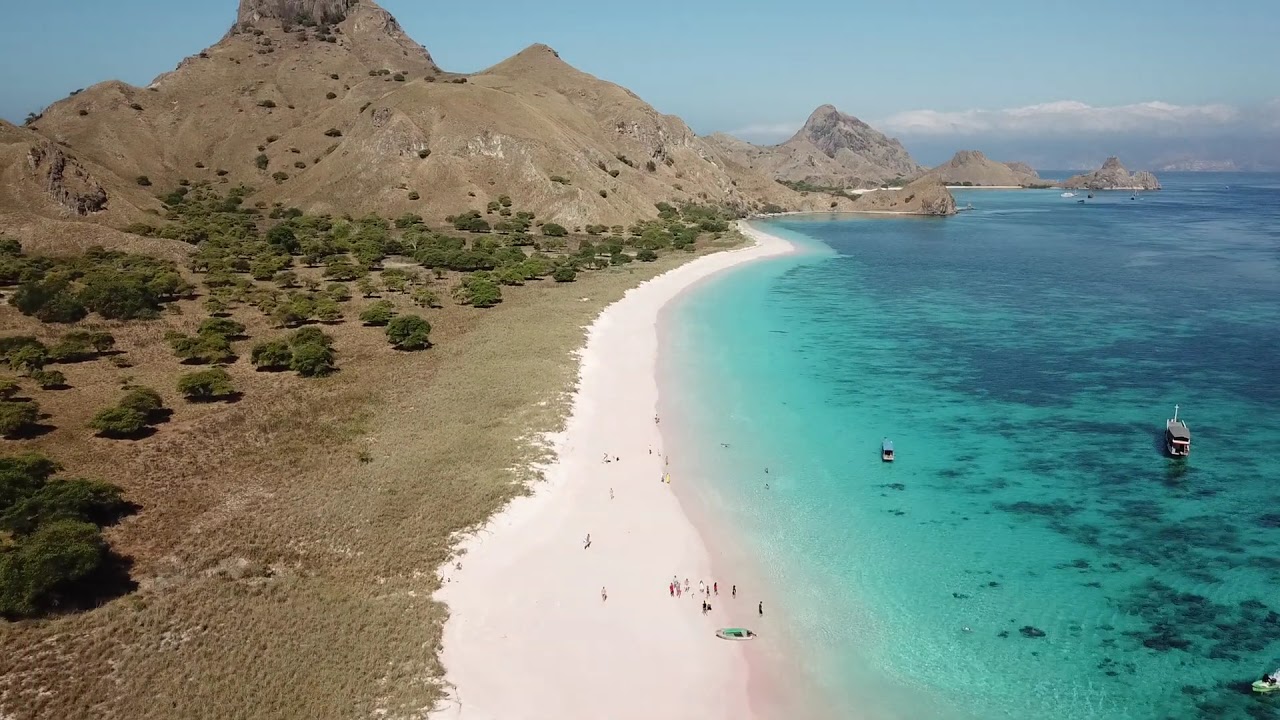In this detailed overhead shot likely taken by a drone, the image captures a curved bay with a stunning white sandy beach stretching through its center. Along the right side, the water is a mesmerizing light blue-green, dotted with darker green patches indicating submerged rocks or vegetation. Scattered across this transparent tropical water are a few thin, tall boats, some appearing black and white.

At the bottom of the image, a significant number of people can be seen converging towards the water, some playing near the shore while others are more spread out along the beach. Notably, there's a small white paddle boat beached nearby. On the left side, dry light brown grass and scattered trees are evident, extending inland up the slope of a majestic mountain range. This range frames the bay from left to right, its large peak dominating the left side of the image and tapering off as it descends towards the water.

Towards the middle of the photo, there is also a distinct walkway populated by numerous individuals. Despite the natural beauty and vivacity of the scene, it is the striking contrast between the clear blue sky, the brownish hues of the mountains and inland foliage, and the vibrant beach activities that encapsulates the vibrant essence of this tropical paradise.